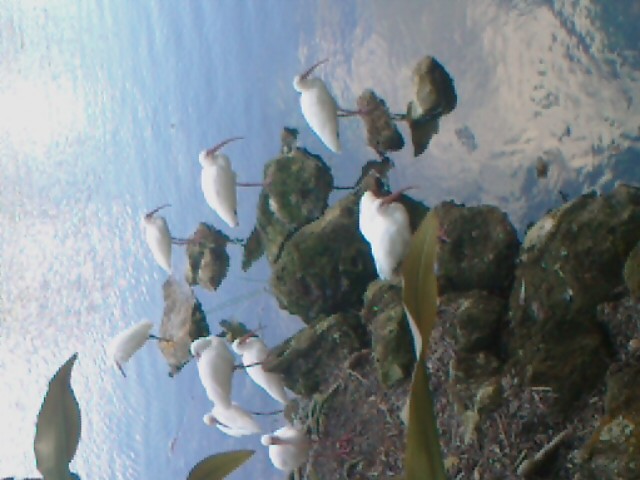This detailed photograph, viewed sideways, captures a serene waterscape featuring a diverse gathering of white, long-legged birds, possibly egrets or cranes, positioned gracefully on and around clustered, moss-covered rocks. There are at least nine birds with strikingly slim, orange beaks and elegant white feathers. The clear blue water, shimmering with reflections of the sun or sky, creates a mesmerizing backdrop. Among the birds, some are perched on individual rocks amidst the water, while others stand on a dirt path behind the rocks, strewn with sticks and leaves. The image includes a few green plant leaves in the foreground, adding depth to the scene. The photo's slight blurriness gives it a delicate, painting-like quality, enhancing its beauty and tranquility.